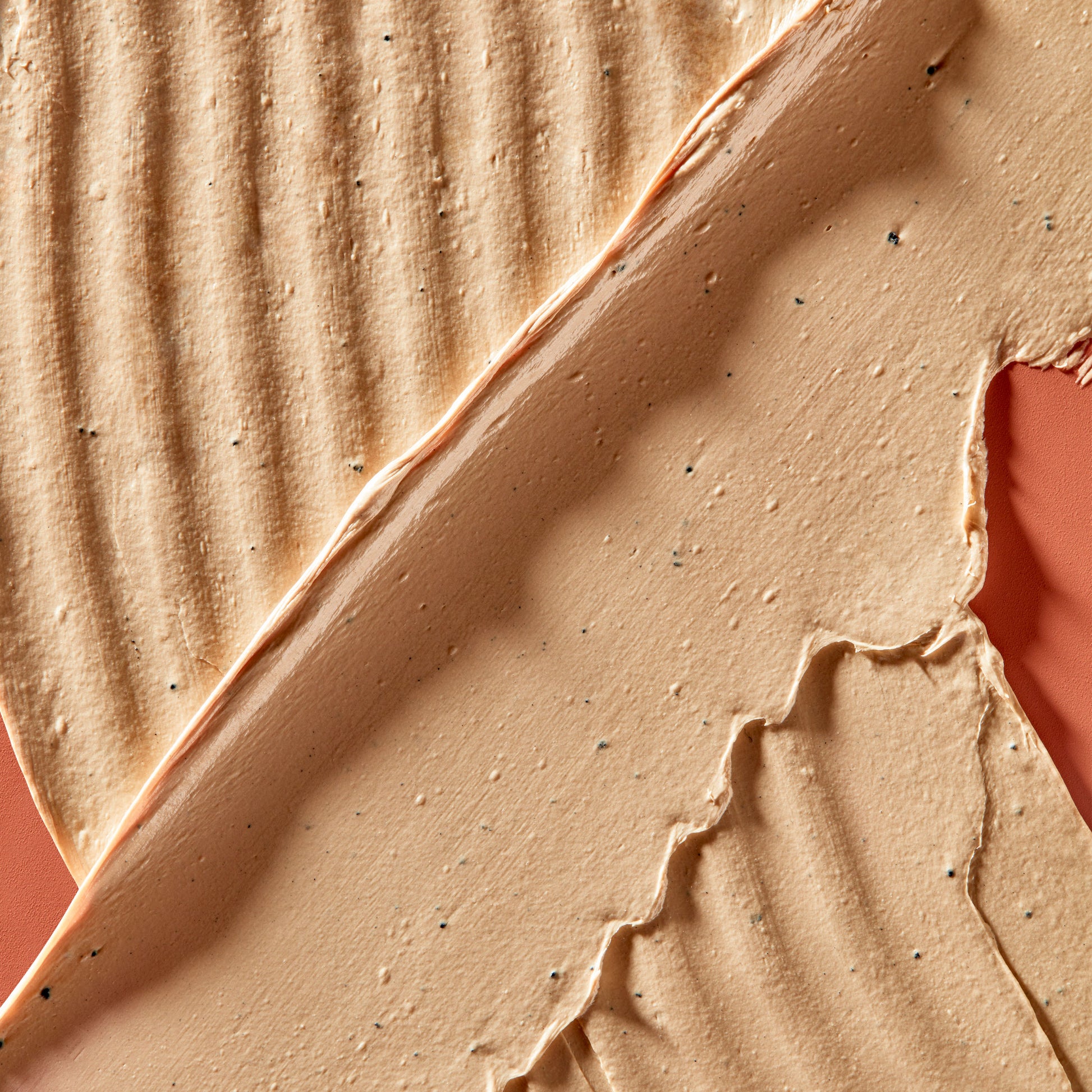This image features a tan brushstroke or layer of frosting that extends from the bottom left to the top right of a square photograph. This foreground brushstroke is thin and appears slightly elevated, casting subtle shadows and adding a three-dimensional aspect to the composition. Below the tan layer, a wider brushstroke with vertical ridges runs from the top left to the bottom right, creating a textured depth. Both layers are laid against a reddish-orange background, emphasizing the contrast and adding warmth to the piece. The gradient of grays on the brushstrokes transitions smoothly from one corner to the opposite, enhancing the overall visual flow and dynamic.